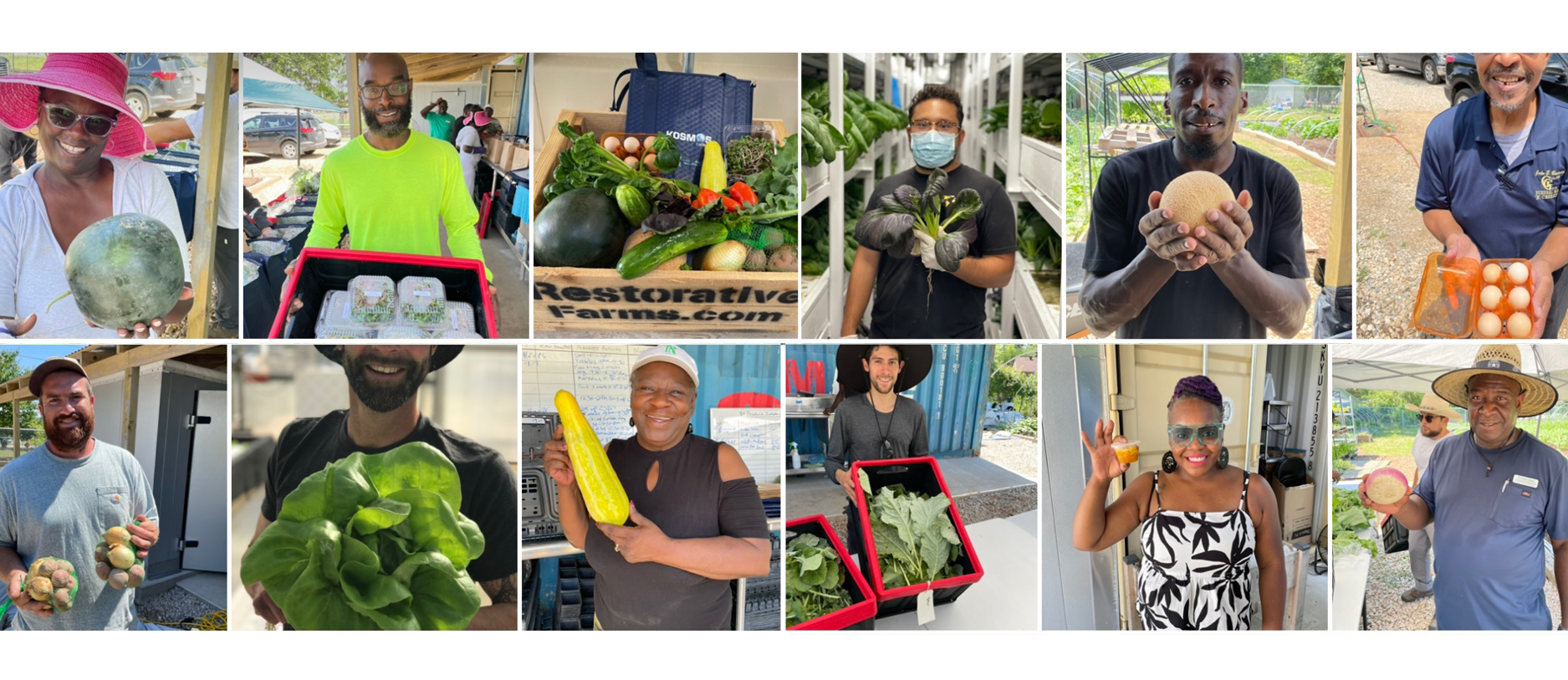This image features a compilation of 12 photographs, arranged in two rows of six, against a white background. Each photo showcases individuals of diverse backgrounds, including Black, White, and likely Hispanic men and women, both inside and outside. Predominantly, they are depicted holding various fruits and vegetables. Notable details include an African-American woman wearing a pink hat and a white blouse, holding a watermelon, and a black man in a yellow t-shirt holding a round fruit. Another individual, a man in a black shirt and bluish mask, is pictured at a vendor stall surrounded by assorted vegetables like lettuce. A cardboard box labeled 'Restorative Farms' with cucumbers and peppers appears in another image. Additionally, a white man with a package of eggs and a lady with yellow squash are among the featured individuals, each proudly presenting their fresh produce or food items.